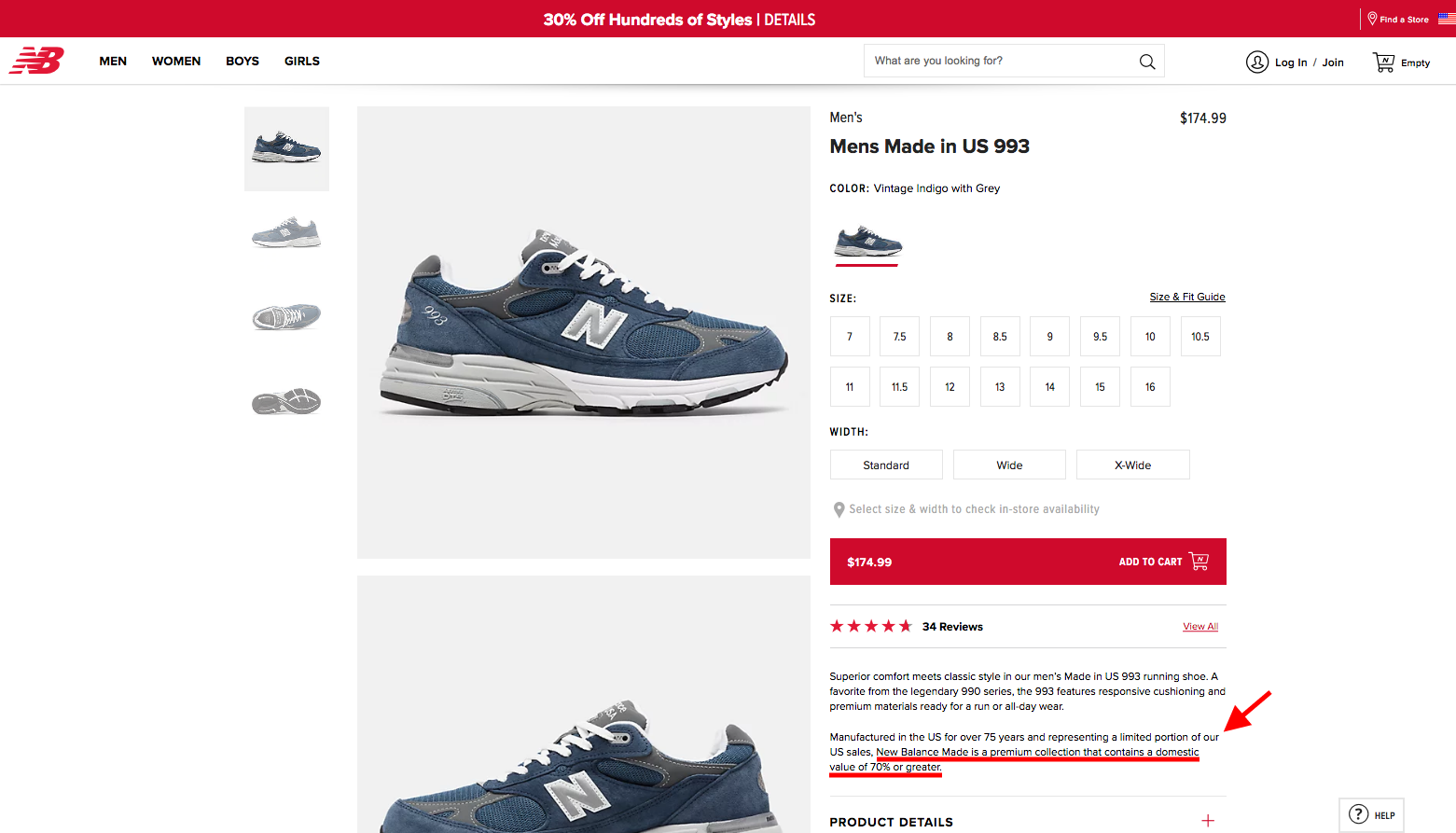In this New Balance website screenshot, the focus is on the Men's Made in US 993 sneaker in the vintage indigo and gray colorway. The central part of the page features a large gray square displaying a prominent image of the sneaker, with a secondary image below showing the sneaker from the opposite direction. To the left of this main box, there are four thumbnail images providing different views of the sneaker. The currently displayed image, with the toe pointing to the right, is on top. Below it, thumbnails include the toe pointing left, an overhead view, and a bottom view, all slightly grayed out to indicate they are not currently selected.

On the right side of the page, there is detailed information about the sizing options. Users can select their desired size and width from interactive boxes, and a prominent red action button allows them to add the sneaker to their cart for $174.99. Below this section, summary information and reviews are provided, showing an average rating of nearly five stars based on 34 reviews. A red "view all" link offers access to all customer reviews.

Further down, descriptive text about the sneaker notes its manufacturing in the US for over 75 years, representing a limited portion of New Balance's US sales. This text features a manually underlined section in red with a hand-drawn red arrow annotation that highlights the sneaker's premium collection status, containing a domestic value of 70% or greater.

At the very top of the screenshot, there is a red banner advertising "30% off hundreds of styles," with a link for more details. The New Balance logo and site navigation menu are also visible in this top section.